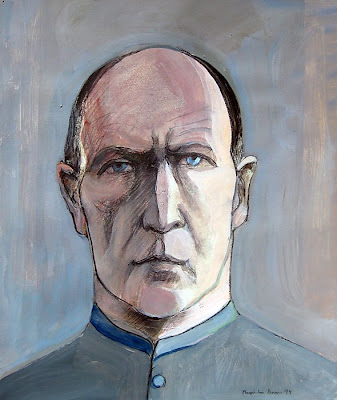The image is a detailed sketch or painting of a man's upper body. The man, depicted with a stern and intense expression, stares straight ahead, his steely blue eyes barely open. His face is elongated and predominantly gray in color, with a touch of flesh tones and redness near his forehead. He has a very receding hairline, leaving most of his scalp bald except for the dark black and gray hair on the sides. His long ears blend into the gray hues of his face.

The man is dressed in a gray suit, which has a high, tight collar. The collar is asymmetrical, appearing darker blue on the left side and more gray on the right, with a single light blue circular button visible just beneath the collar on the right side. The background is a smudged mix of gray and light blue, enhancing the seriousness of the portrait. There is a small, indecipherable black cursive signature in the bottom right corner of the image. Overall, the portrait's style combines elements of sketching and painting, creating an intriguing and stark visual effect.